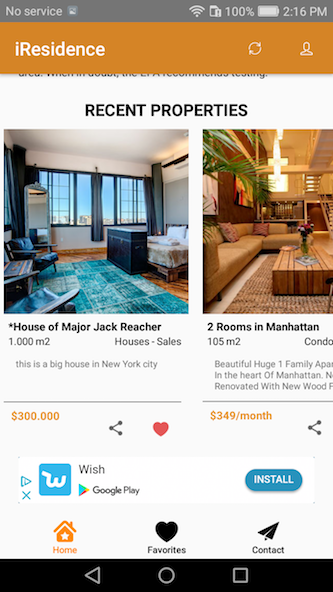The image appears to be a screenshot of a mobile-optimized real estate website. The interface has several distinct sections and visual elements:

- **Top Bar**: 
  - A grey band displays system information. To the left, "No Service" is indicated in white text. To the right, a full WiFi icon, a 100% battery indicator, and the time, 2:16 PM, are visible.
  
- **Header**:
  - Below the top bar, an orange band with the text "iResidence" appears. On the right side of the band, there are two icons: one circular and the other depicting a person’s head.
  
- **Main Content**:
  - The background here is white. Centered text reads "Recent Properties" in black.
  - There are two displayed property listings:
    1. **Left Listing**:
       - Displays a property with grey walls and a blue-themed interior.
       - Includes a visible blue window, a blue rug on a wooden floor, and a blue press or table. Possibly a bed in the background, but it's too small to distinguish clearly.
       - Title: "House of Major Jack Reacher"
       - Details: 100 M², 1002 house sales, located in New York City.
       - Price: Highlighted in orange, $300,000.
       
    2. **Right Listing**:
       - Resembles a hotel room.
       - Shows a couch, a coffee table, a plant, beige-orange walls, and a beige carpet.
       - Title: "Two Rooms in Manhattan"
       - Details: 105 M², with partial additional text reading "beautiful, huge seven family in the heart of Manhattan, renovated with New York."
       - Rental Price: $349 per month, highlighted in orange.
       
- **Ad and Navigation Bar**:
  - An ad for an app available on Google Play, featuring a "Whoosh" button.
  - Navigation icons at the bottom feature three white icons on a black band: a back icon, a home icon, and a square icon for recent apps.

Overall, the layout is clear and user-friendly, providing quick access to property details and prices within a well-structured mobile interface.